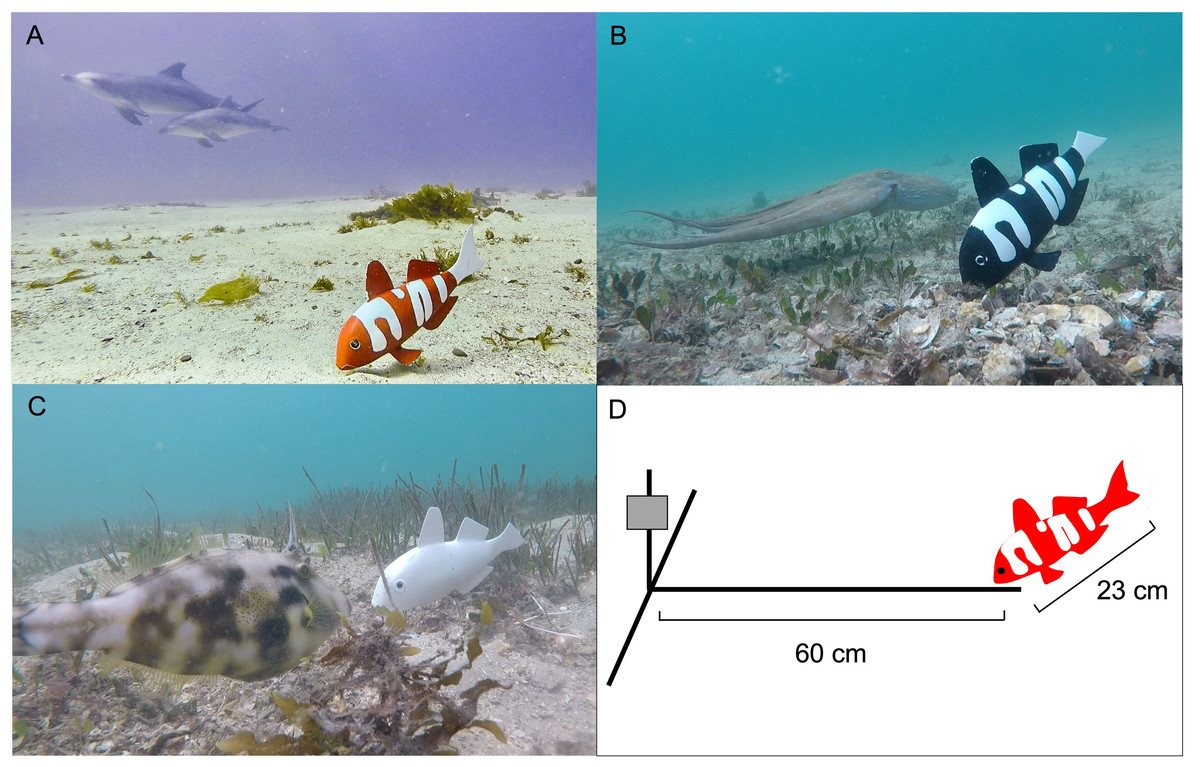This poster features four distinct squares labeled A, B, C, and D that combine photographs and illustrations. In square A, located in the upper left, a computer-generated scene depicts an underwater environment characterized by a sandy bottom with sparse seaweed. Here, an orange and white striped fish is seen navigating the seabed while a larger fish looms in the background. Square B, positioned in the upper right, presents another aquatic setting, this time with a rocky bottom and bluer aquamarine water. It showcases a black and white fish, possibly generated through digital means, interacting with the environment, alongside what appears to be a squid or stingray. Square C, found in the lower left, features a sandy and seaweed-dotted seabed under blue ocean water. This image includes an albino-like white fish and another camouflaged, possibly brown and white fish, both sharing a resemblance to goldfish in their body shape. Lastly, square D in the bottom right corner diverges from the photographic theme, presenting a technical line drawing. This diagram measures an orange and white fish's path, indicating a 23-centimeter descent and a straight 60-centimeter horizontal stretch, likely providing context for the size and placement of the fish in the other images. The composition blends detailed underwater photography aesthetics with schematic illustrations to offer a cohesive and informative visual narrative.